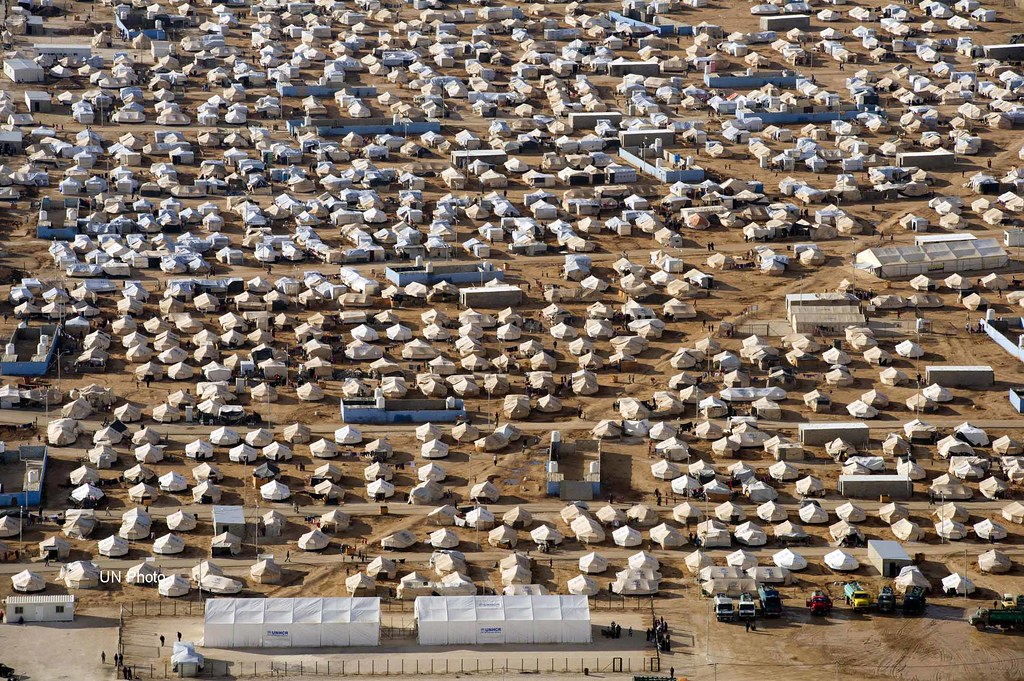The image captures a high-altitude view, possibly from an airplane or satellite, of a large camp in a barren, brown dirt field. The camp is meticulously organized, featuring rows of small white tents that extend from the bottom to the top of the image, numbering around one to two hundred. At the bottom and forefront of the image, two larger white rectangular tents are enclosed by a black fence, surrounded by a collection of approximately six parked trucks. Further into the camp, amidst the smaller tents, are scattered blue buildings and additional larger white structures. These facilities appear to be centrally located among the sea of smaller tents and continue to dot the landscape into the background.